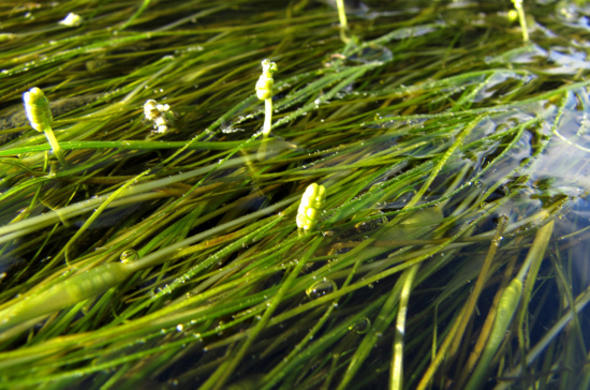This detailed, full-color photograph, taken in landscape orientation during the daytime, captures a nature scene of aquatic vegetation. The image predominantly showcases seagrass lying flat and extending diagonally across the water surface, creating a lush green expanse. The thin blades of grass stretch from the top to the bottom and across the entire width of the image, giving it a sense of dense, uninterrupted greenery.

In addition to the main greenery, several thin stalks rise vertically from the water, each topped with tiny, round, greenish-yellow buds that resemble miniature peas. These small sprouts vary in size and shape, adding a layer of texture and depth to the scene. The clear water reveals subtle reflections, particularly on the upper right, capturing light that contrasts with the darker tones of the water seen in the bottom right corner. Bubbles are sporadically visible, adding to the realism and dynamic nature of this vibrant, realistic representation of underwater flora.